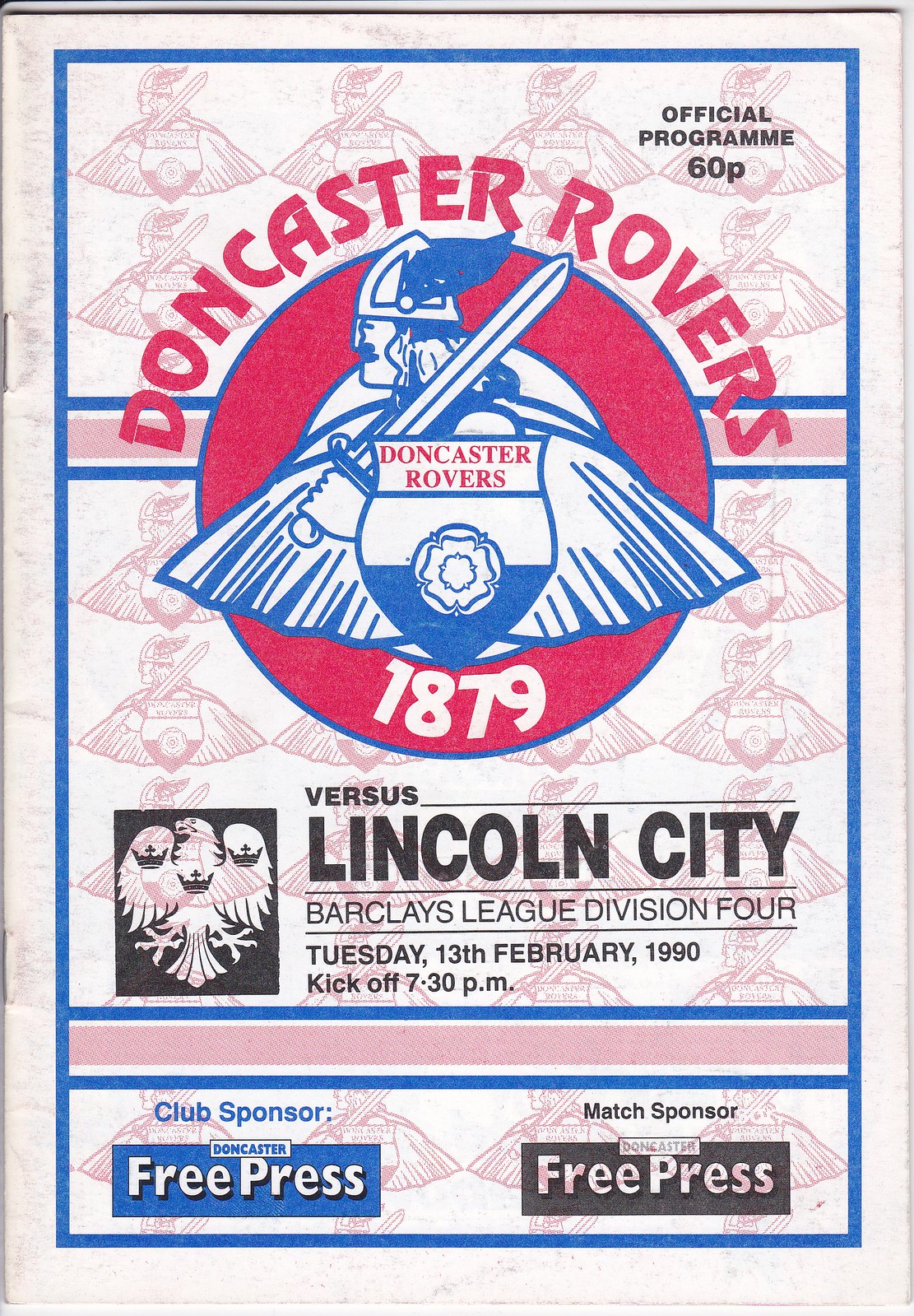The image displays the front cover of an official program for a football match. At the top, it prominently features the title "Doncaster Rovers" along with a logo depicting a warrior or knight wearing a helmet and holding a sword, with the year "1879" inscribed. The program details a match between Doncaster Rovers and Lincoln City, taking place in the Barclays League Division IV on Tuesday, 13th February 1990 at 7:30 p.m. 

A distinctive logo of an eagle adorned with three crowns (one on each wing and one in the middle) is also present. The words "Official Program" are located in the upper right corner. Notably, the program is sponsored by the Doncaster Free Press, with both the club and the match sponsors being mentioned at the bottom. The color palette includes blue, white, pink, black, gray, red, and maroon, and the entire cover exudes the feel of an official match-day memorabilia item.